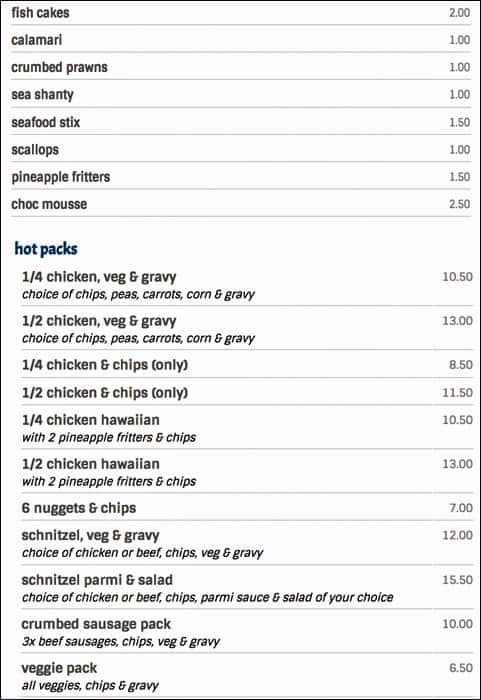The image features a menu list for a seafood restaurant, presented in a rectangular format with a white background and a thin black outline. The menu is organized with items left-justified and their corresponding prices right-justified, separated by horizontal gray lines. The listed items include:

- Fish cakes: $2.00
- Calamari: $1.00
- Crumbled prawns: $1.00
- Sea shanty: $1.00
- Seafood sticks: $1.50
- Scallops: $1.00
- Pineapple fritters: $1.50
- Chocolate mousse: $2.50

Below this section, "Hot Packs" is highlighted in blue font, while the rest of the text remains in black:

- Quarter chicken, vegetables, and gravy with a choice of chips, peas, carrots, corn, and gravy: $10.50
- Half chicken, vegetables, and gravy with a choice of chips, peas, carrots, corn, and gravy: $13.00
- Quarter chicken and chips only: $8.50
- Half chicken and chips only: $11.50
- Quarter chicken Hawaiian with two pineapple fritters and chips: $10.50
- Half chicken Hawaiian with two pineapple fritters and chips: $13.00